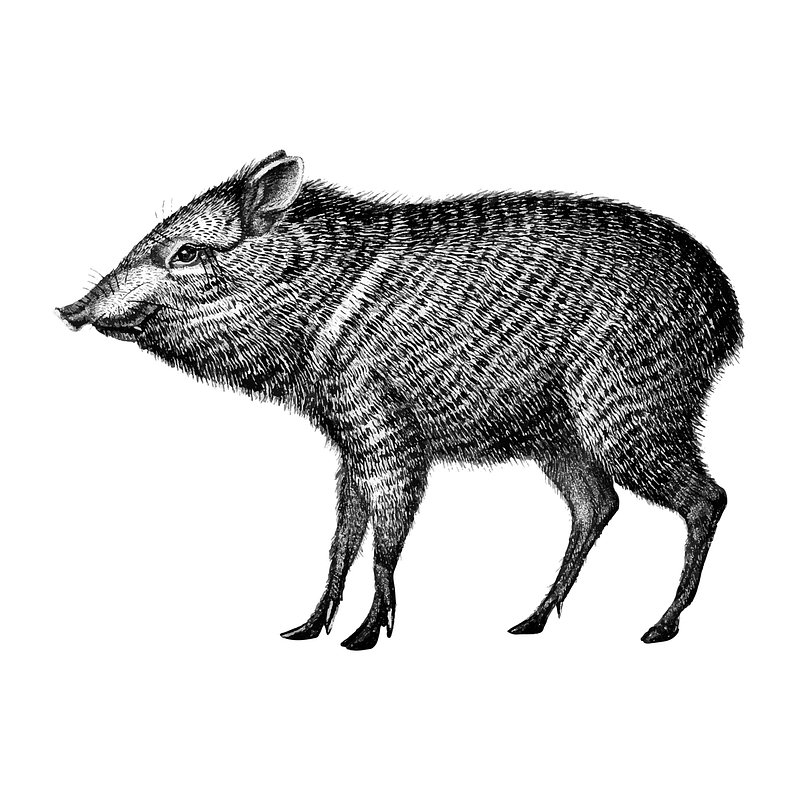This black and white illustration, likely done in ink on white paper, depicts a side view of a small, furry boar. The animal is detailed with fine, tiny strokes capturing its coarse, textured fur, which includes some darker striations. It has a pig-like snout, small ears, and piercing dark eyes. Its legs are spindly and end in tiny hooves, with what appear to be small, spike-like nails beside each hoof. The boar's head and neck are of similar width, and if it has a tail, it is very small and inconspicuous. Overall, this hand-drawn piece showcases a meticulously detailed rendering of the boar, highlighting every hair and feature with precision.